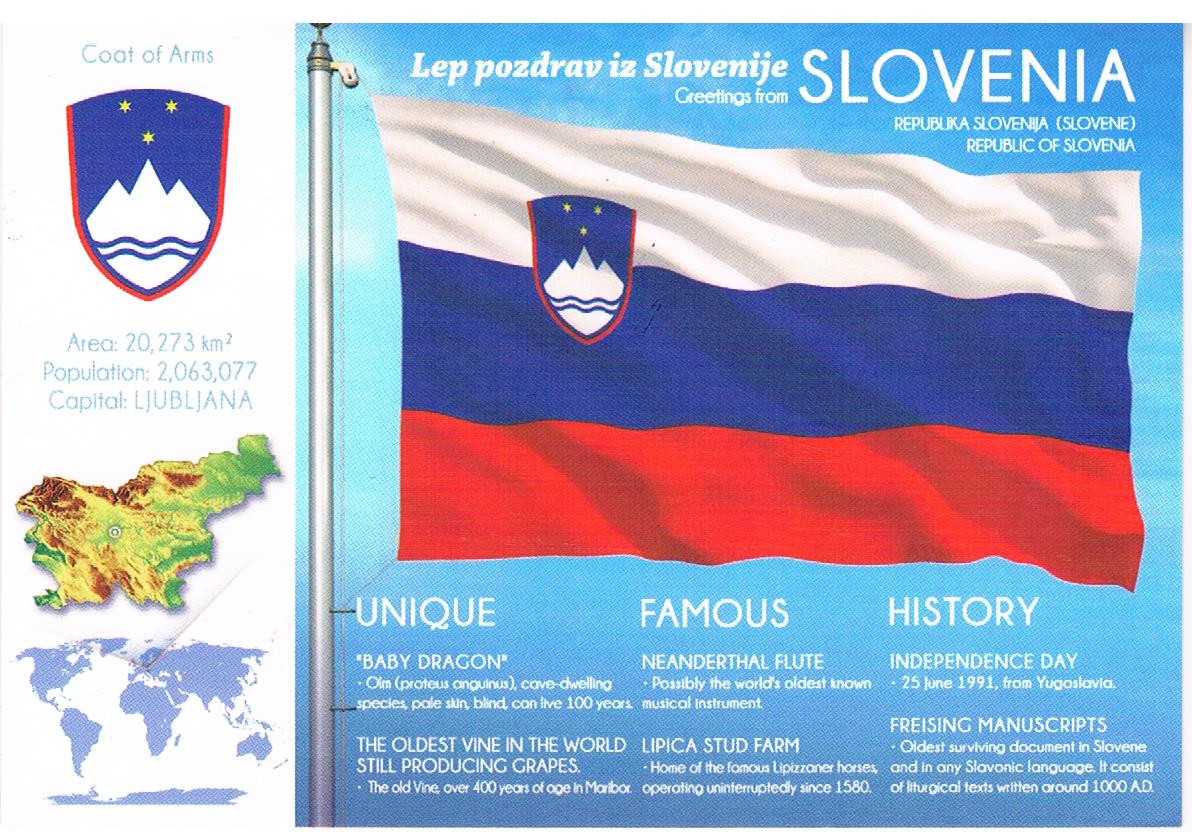This horizontally aligned rectangular image primarily highlights the flag of Slovenia on the right. The flag is held up by a large silver pole and consists of three horizontal stripes: white at the top, blue in the middle, and red at the bottom. Above the flag, in large all caps white letters, it says "LEP POSDRAV EZ SLOVENIA" which means "greetings from Slovenia." Below this, it reads "Republika Slovenia" followed by "Republic of Slovenia" in parenthesis. At the bottom right, there are three bolded headings: "unique," "famous," and "history," each accompanied by descriptive text elaborating on Slovenia's distinct features, notable facts, and historical details. To the left of the flag, there is a white vertical section featuring a coat of arms badge outlined in red, depicting a white mountain with stars above it on a blue background. Below this badge, text specifies Slovenia's area as "20273 square kilometers," its population as "2063077," and its capital as "LJUBLJANA." Further down, there is a small map of Slovenia in brown, light brown, and green, followed by a world map in white and blue indicating Slovenia's location on the continents. The overall aesthetic suggests the image might be part of a larger presentation slide deck.